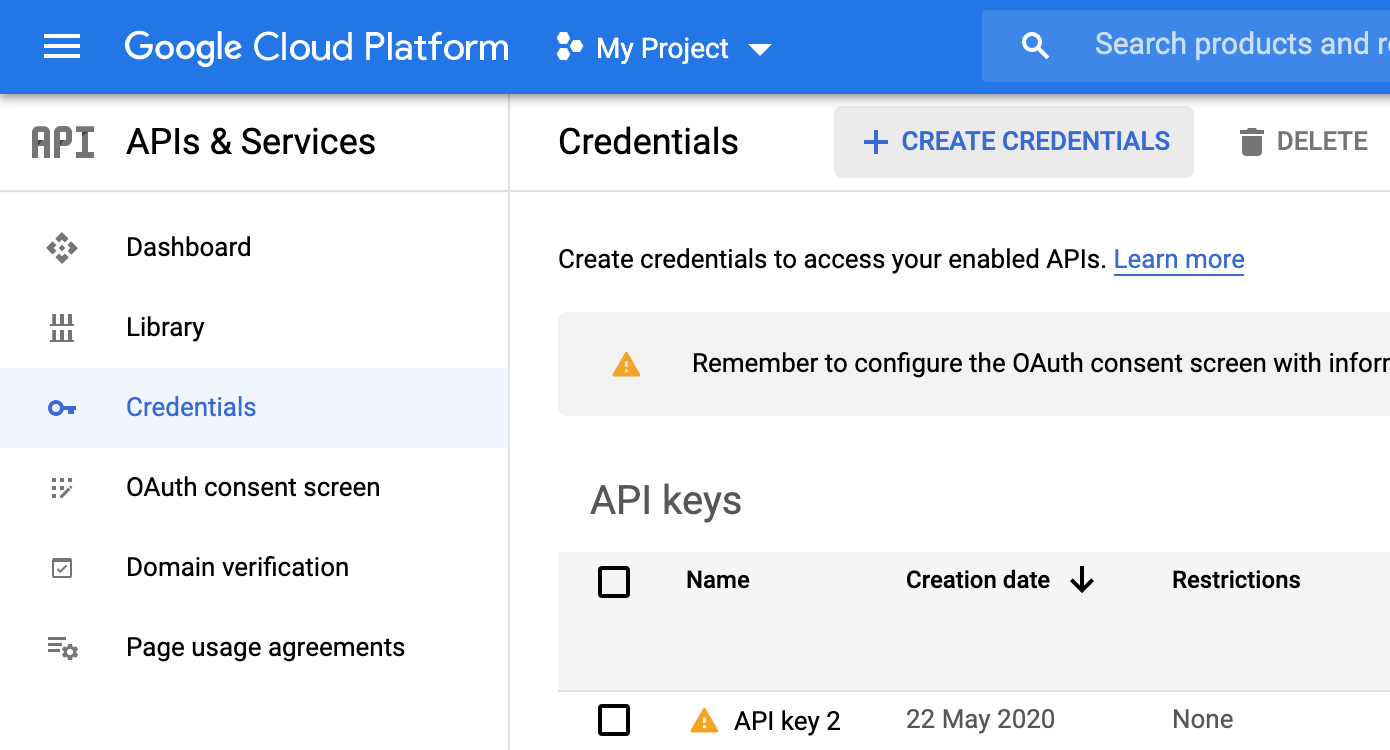The image shows a detailed interface of the Google Cloud Platform, predominantly displaying the "Credentials" page under the "API & Services" section. At the top, the screen features a blue border, with the Google Cloud Platform logo on the upper left-hand corner. Adjacent to the logo, a hamburger menu icon consisting of three horizontal white lines is visible beside a "My Project" drop-down menu.

Further below, a slightly lighter blue bar provides a search field labeled "Search Products." The image is partially cut off at this point. Beneath this blue section, the main interface showcases a clean white background with the section header "API & Services" prominently displayed in black font. Sub-sections beneath this header include clickable options such as Dashboard, Library, Credentials, OAuth Consent Screen, Domain Verification, and Page Usage Agreements.

Currently, the "Credentials" sub-section is highlighted in blue, indicating it is the active page. On the right-hand side of the screen, the "Credentials" interface is open, displaying relevant controls and information. There is a blue button labeled "Create Credentials" along with a trash can icon for the delete function beside it. The instructions beneath this button read, "Create credentials to access your enabled APIs, learn more. Remember to configure the OAuth Consent Screen with..." and the text cuts off here.

Additionally, the page lists credential details including "API keys" along with their respective "Name," "Creation Date," and "Restrictions." An example entry shows "API Key 2" with a creation date of "22 May 2020" and indicates that there are "no restrictions." The displayed content and design emphasize user control and clarity within the credential management interface of the Google Cloud Platform.